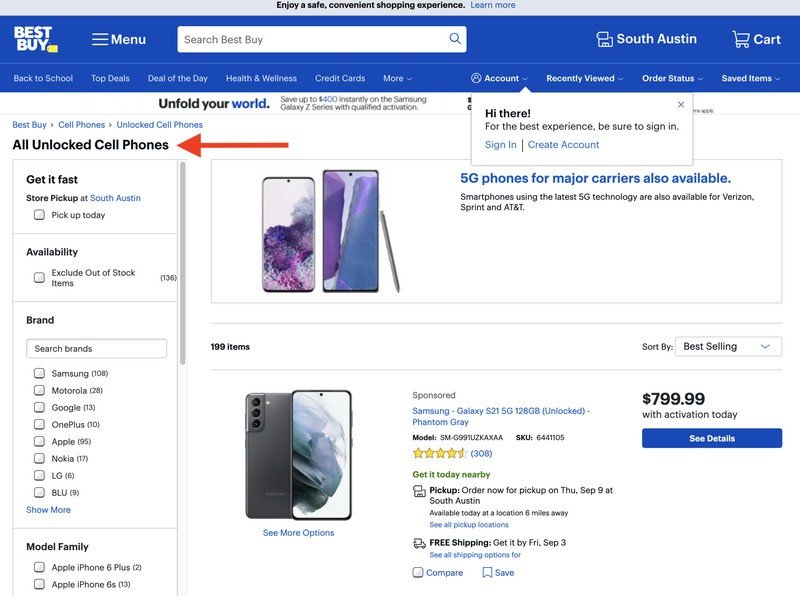The image is a detailed screenshot of Best Buy's product listing page for unlocked cell phones, clearly marked by the prominent Best Buy logo in the top left corner and accompanied by a comprehensive menu bar. The menu bar includes multiple links such as "Back to School," "Top Deals," "Deal of the Day," "Health and Wellness," "Credit Cards," and more. A functional search bar with the placeholder "Search Best Buy" is prominently displayed.

To the right of the search bar are user navigation options: Account, Recently Viewed, Order Status, and Saved Items. The store location is specified as South Austin, and there is a cart icon showing an empty cart. Beneath the navigation, a breadcrumb trail displays the navigation path: Best Buy > Cell Phones > Unlocked Cell Phones > All Unlocked Cell Phones, with "All Unlocked Cell Phones" highlighted by a red arrow.

A promotional banner states, "Unfold your world: Save up to $400 instantly on the Samsung Galaxy Z series with a qualified activation." There is also a sign-in prompt saying, "Hi there, for the best experience be sure to sign in," with options for signing in or creating an account. Another promotion announces the availability of 5G phones for major carriers.

On the left sidebar, filters allow for customization of search results, including "Get it fast" with store pickup at South Austin, and options to pick up today. Filters also allow users to exclude out-of-stock items, showing that 136 items are available. Brand filters reveal counts of phones per brand: Samsung (108), Motorola (28), Google (13), OnePlus (10), Apple (9), Nokia (8), LG (6). Model families include listings like Samsung Galaxy Note 8, Samsung Galaxy S7, and Apple iPhone 11.

The main product listing area shows 199 items. The listing can be sorted using a dropdown box with "Best Selling" as an option. The specific product shown is the Samsung Galaxy S21 5G, 128GB, in Phantom Gray. Detailed specifications include model number and SKU (SM-G991UZKAXAA, SKU: 6441105), with a rating of 4.4 stars based on 308 reviews. The price listed is $799.99 with activation today. Availability options include in-store pickup by Thursday, September 9th at South Austin or free shipping by Friday, September 3rd.